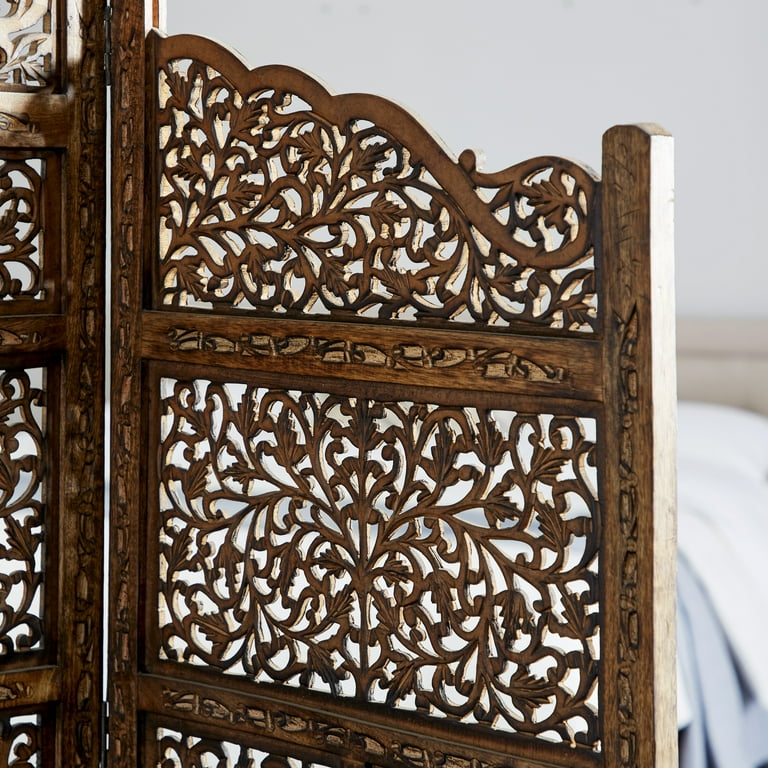In the foreground of the image, there is an ornate wooden folding room divider composed of two visible panels connected by metal hinges at the top and bottom left corners. The divider is intricately designed with dark and light wood, showcasing detailed floral and vine patterns. These designs are carved into the wood, with sections cut out between the vines and flowers, allowing you to see through the panels. The borders of the panels are solid wood, and the top features a wavy curve with a thicker vine design. In the background, a spacious bedroom is visible, highlighting a large bed adorned with white sheets, a blue comforter, and a gray fabric headboard. The wall behind the bed is painted a light gray, complementing the serene, rustic ambiance of the scene.